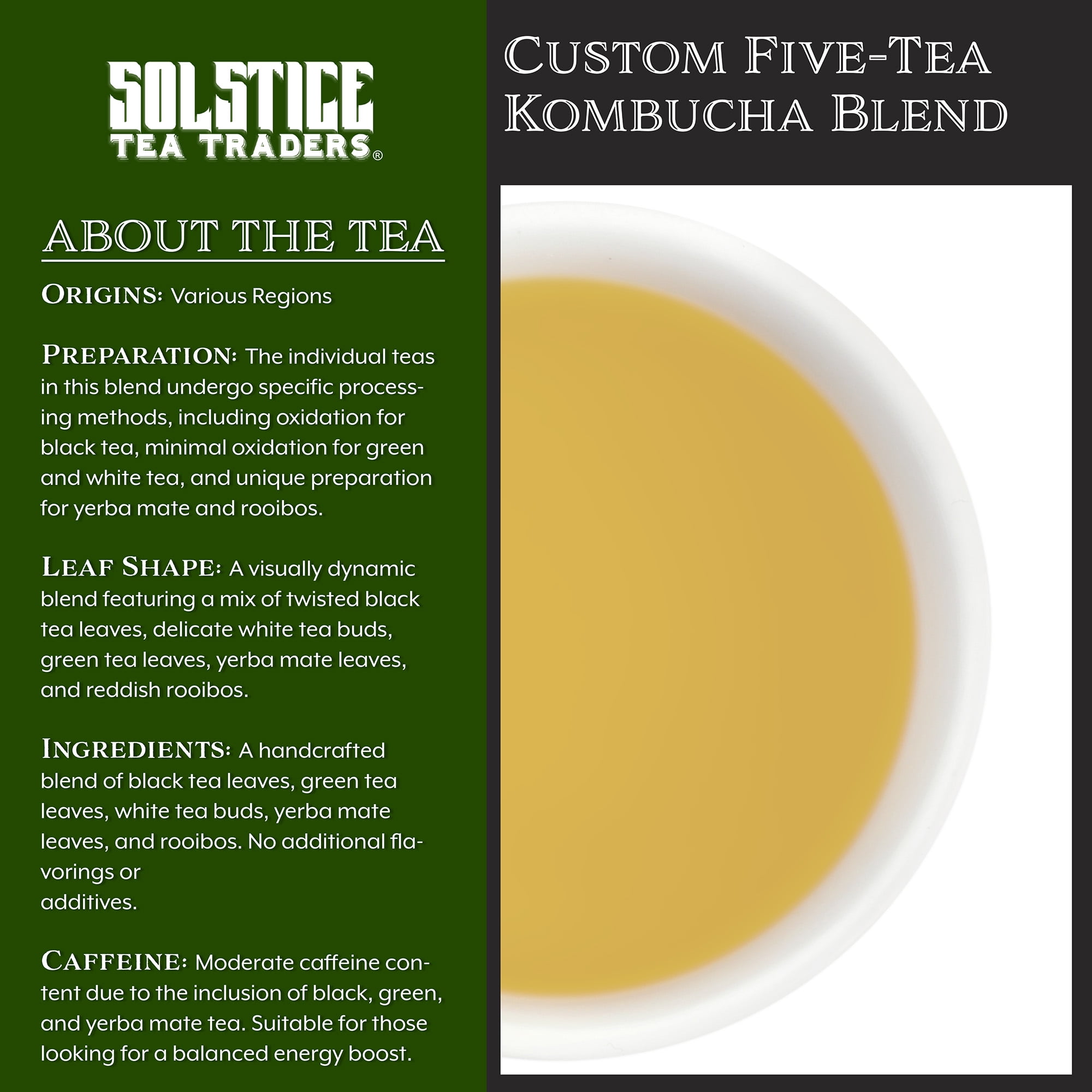This image is an advertisement for a custom 5 tea kombucha blend by Solstice Tea Traders. It features a split design with the right side displaying a bird’s eye view of a teacup filled with light yellow tea on a white background. Above the teacup, in white serif font on a black background, are the words “Custom 5 Tea Kombucha Blend”. The left side of the image has a dark green background accentuated with white text detailing the product information. At the top, it prominently reads “Solstice Tea Traders”. The text below this heading provides an in-depth description of the tea, including origins from various regions, preparation methods such as oxidation for black tea and minimal oxidation for green and white tea, and unique preparations for yerba mate and rooibos. The tea blend features a visually dynamic mix of twisted black tea leaves, delicate white tea buds, green tea leaves, yerba mate leaves, and reddish rooibos. The ingredients comprise purely handcrafted elements with no additional flavorings or additives. Lastly, it highlights the moderate caffeine content, offering a balanced energy boost due to the inclusion of black, green, and yerba mate teas. The overall style of the ad is modern, emphasizing detailed product descriptions alongside the aesthetic appeal of the tea.